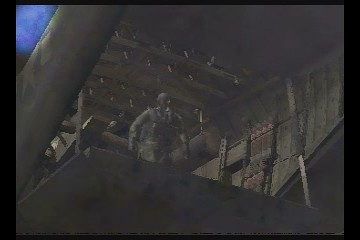The image depicts a suspenseful moment within a video game, captured from a midair vantage point, focusing on the interior of an open cargo plane. The cargo door is wide open, revealing a man standing at the edge of the doorway, either poised to jump or looking out at the vast expanse behind him. Surrounding him, the interior walls are lined with various objects, possibly parachutes, secured in place. The mechanical hydraulic arms are visible, holding the cargo door firmly open, adding an element of mechanical realism to the scene. At the top of the cargo bay, ominous spikes protrude from the ceiling, contributing to the tension and perhaps hinting at an underlying danger. The dim lighting envelops most of the scene in shadow, though in the upper left corner, a glimpse of a clear blue sky provides a stark contrast to the otherwise dark atmosphere.